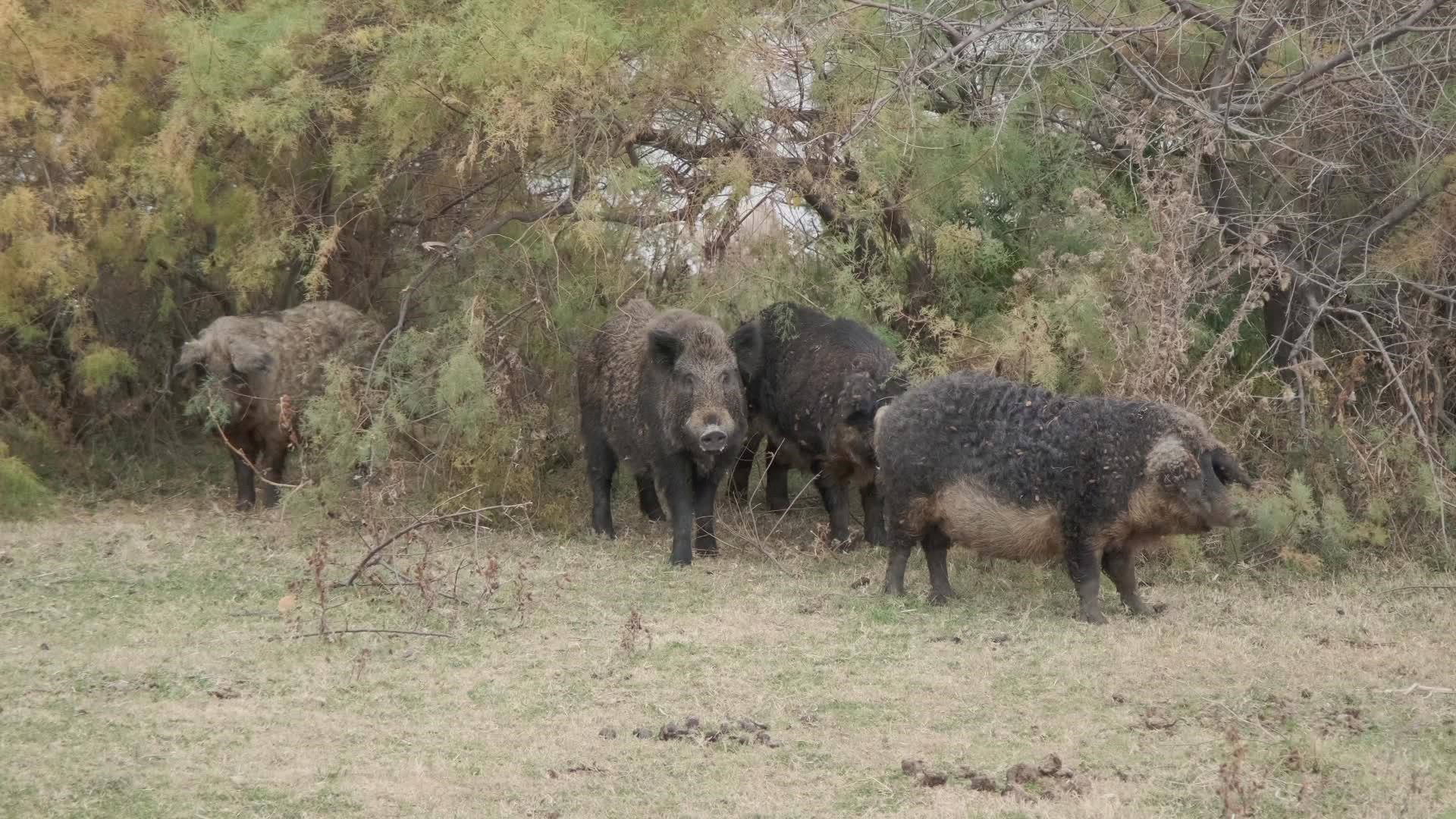This photograph captures a group of four wild pigs in a natural outdoor setting, presenting a vivid scene of untamed wilderness. The pigs, which showcase a mix of black, dark gray, and brown fur, are prominently positioned against a backdrop of low green and brown trees. Their fur appears darker on their backs and legs, transitioning to lighter shades on their underbellies and faces, and they are covered in debris like tree pieces and dirt, adding to their rugged appearance. The pigs are all facing the camera, with only one not fully visible. They walk amidst a landscape characterized by dry, tan-colored grass and scattered sticks, blending seamlessly with the scrub environment. The sky is a clear blue beyond the treetops, contributing to the daylight illumination of the scene. The photograph effectively captures the essence of these wild pigs in their natural habitat, emphasizing their earthy, untamed demeanor.